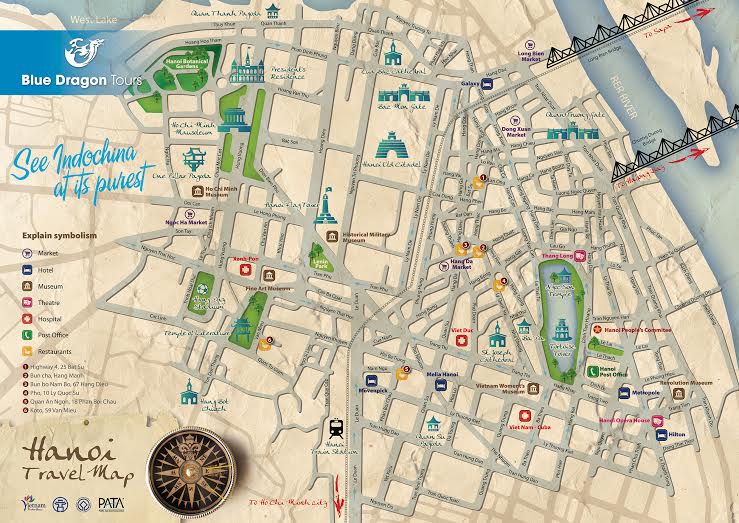This image depicts a detailed and informative Hanoi travel map. The top left corner features a blue rectangular banner with the text "West Lake Blue Dragon Tours" and an icon, followed by the phrase "See Indochina at its purest" in blue cursive. Below this is a comprehensive map key that explains various symbols: a shopping cart for market, a bed for hotel, a building for museum, dramatic masks for theater, a cross for hospital, a phone for post office, and an indiscernible symbol for restaurants. The map itself shows beige land areas, blue waterways including the prominent Ruhr River, gray streets, and green parks. At the bottom left corner, the words "Hanoi Travel Map" are visible alongside an old-school compass with black and bronze details. The map is crisscrossed with streets, labeled with the names of various landmarks; two black bridges span the river, connecting different parts of the city, enhancing the utility of the map for tourists. The overall design suggests a practical tool for exploring the Hanoi area, showcasing its significant buildings and recreational spots.